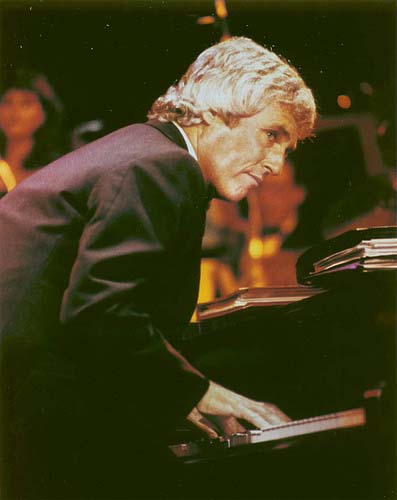This tall, rectangular photograph captures a moment of intense concentration as a piano player leans over his instrument, his body bent down as he faces the right. The pianist, wearing a black suit with a hint of a white collared shirt underneath, has long, blonde, almost whitish hair that reflects the light. His hair is somewhat long, covering his ears, and his head is mostly in profile, with his gaze directed slightly forward.

The piano is situated in the bottom right corner of the image, with an upper shelf above the keys bearing two thick composition books, likely holding his own musical notations. The musician's hands rest on the piano keys, indicating his engagement with the instrument.

In the background, the scene becomes more complex, with blurred figures adding depth to the composition. In the top left corner, a blurry image of a woman with dark brown hair can be seen, while towards the right side, another blurred figure appears to be a man in a suit, possibly playing an instrument. Both background figures contribute to the ambiance without detracting from the central focus on the pianist.